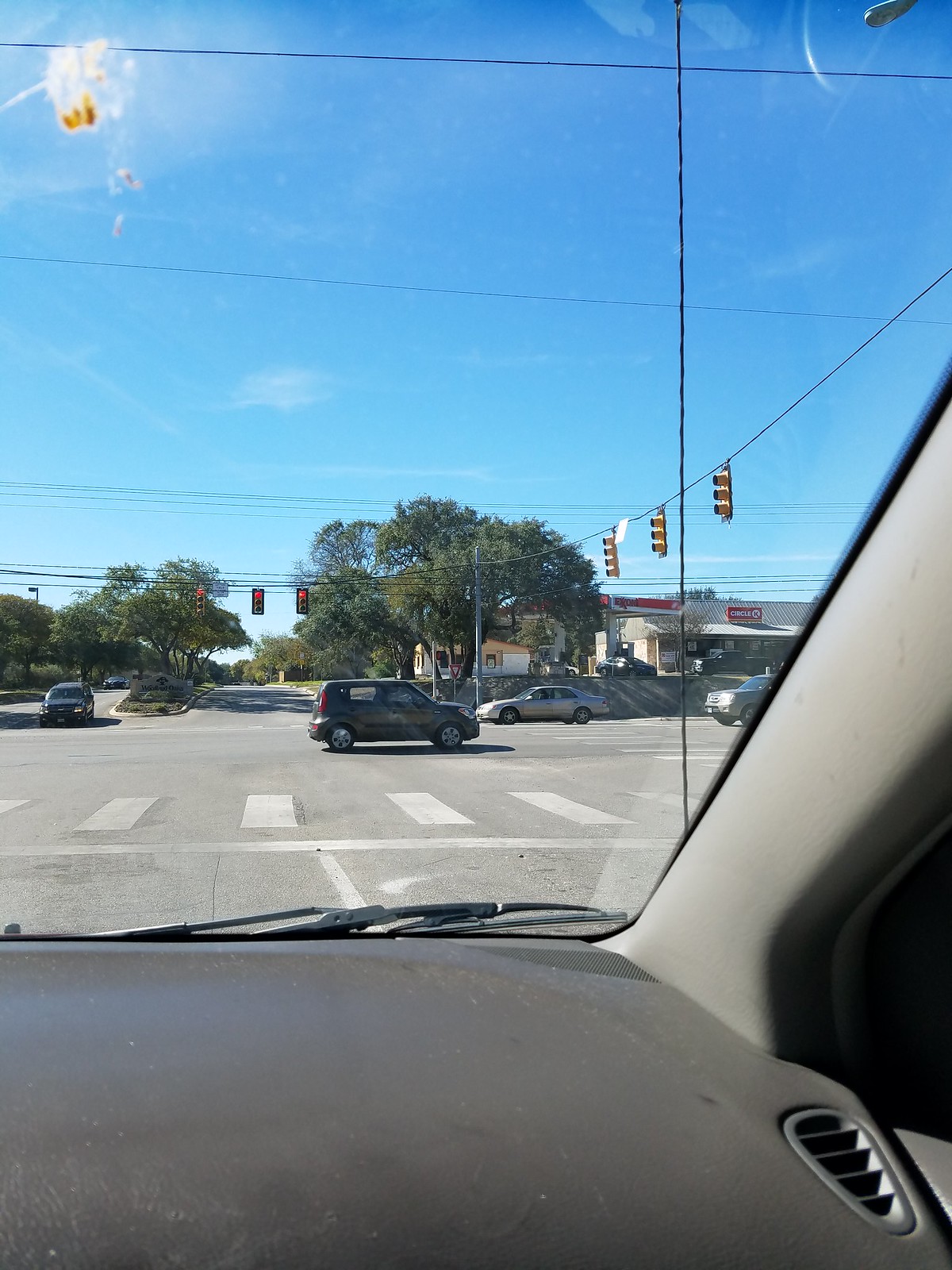This photograph, captured from the passenger side of a car in the United States, offers a detailed view through the windscreen. The bottom right corner of the image displays the car's gray dashboard featuring a passenger air vent, with the light gray inner lining of the car frame also visible. Along the bottom edge, where the glass meets the plastic, the windscreen wiper can be seen resting outside.

The primary focus of the photograph is an intersection ahead. The sky above is a gradient of deep blue at the top, transitioning to pale blue and almost white near the horizon. Suspended on a wire in front of you are three traffic lights, all glowing red, signifying a stop. Perpendicular traffic, moving from left to right, is likely guided by green lights from another set of suspended traffic lights. The top left corner of the windscreen is marred by a small bird dropping. Below, on the gray asphalt, a pedestrian crossing is clearly marked. The overall scene paints a vivid picture of an urban intersection paused in the midst of activity.